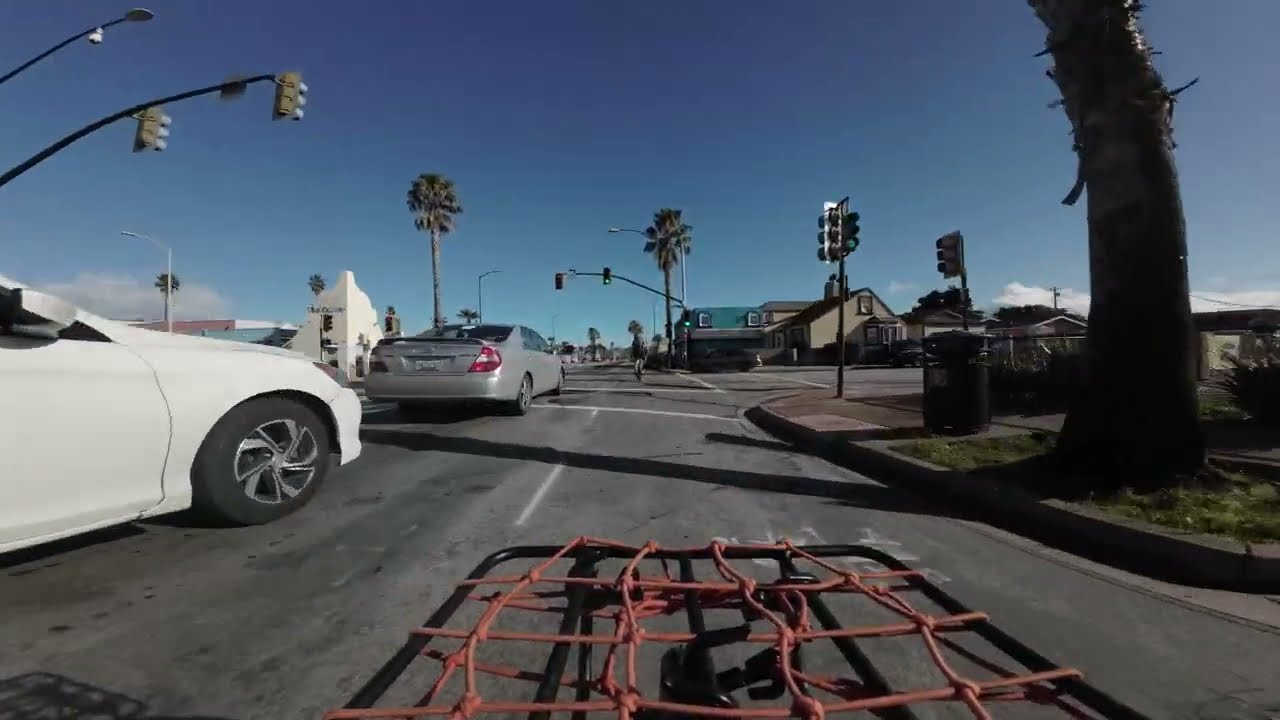Captured from the perspective of a GoPro camera mounted on a bicycle, this image showcases a clear, sunny day on a bustling city street, possibly somewhere in the western United States like Los Angeles. The cyclist is navigating a four-way intersection with a green light, positioned in the far-right bike lane. Just ahead in the same lane is another bicycle approximately 100 feet away. 

To the left of the cyclist are two cars: a white sedan followed by a gray sedan, both moving in the same direction. Prominently visible is a black-framed trailer with an orange rope tied in a grid pattern, situated directly in front. In the middle of the road and to the sides of the street are several palm trees, with one tall palm stalk distinctly close to the camera's frame. 

The background features a mix of small buildings and houses, some of which possibly serve as restaurants. Notable buildings include a uniquely shaped white structure with a slanted façade, alongside other structures painted green and tan. Additional details include a sidewalk running along the street, a garbage can on the side of the road, and traffic lights that point in the opposite direction appearing at the top left of the image.